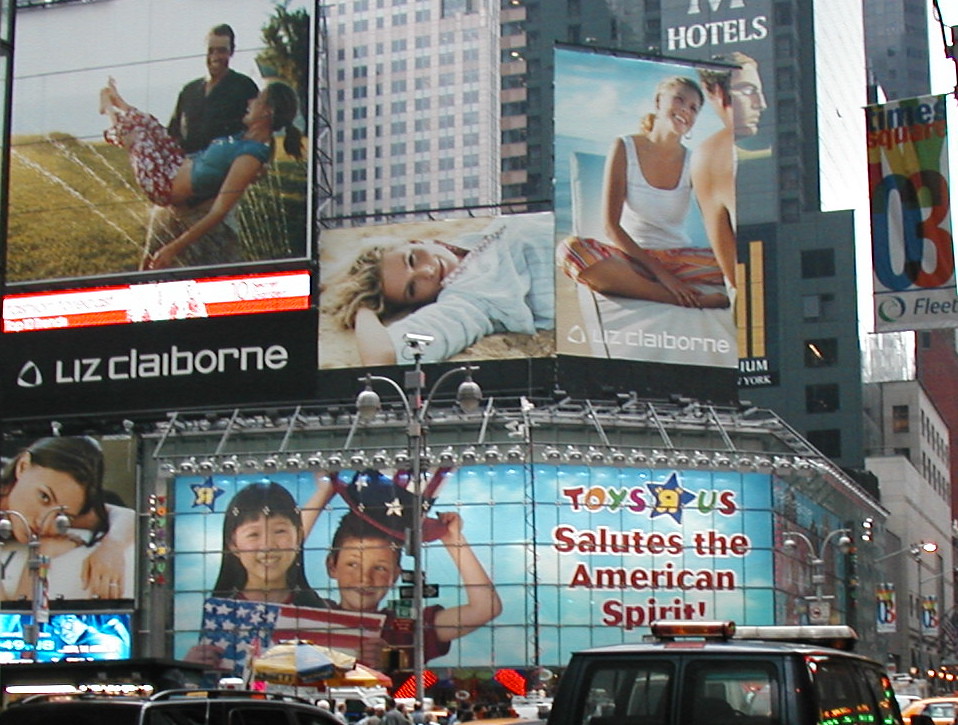The photograph captures a bustling cityscape adorned with a variety of vibrant billboards. Prominently displayed is an advertisement featuring a serene scene of a woman seated cross-legged on a beach, clad in a white tank top and shorts, exuding a sense of tranquility. Adjacent to this, another billboard displays a woman reclining on the sand, wearing a long-sleeved shirt with the sleeves casually rolled up, contributing to the relaxed beach theme.

To the left, a striking image shows a man in a black shirt and tan pants embracing a woman dressed in a blue shirt and red pants adorned with white flowers. This couple stands in a verdant field of grass, emphasizing a sense of freedom and connectedness. Below this scene is the iconic branding of Liz Claiborne, followed by another visual of a woman laying on her hands, perhaps a continuation of the fashion theme.

On the right side of the image, a large and nostalgic sign proudly declares, "Toys R Us salutes the American spirit." This billboard, evidently from a bygone era, features an Asian child holding an American flag beside a white child donning a patriotic top hat, symbolizing unity and national pride. The imagery and slogans reflect a period when such expressions were commonplace, adding a historical layer to the photograph.